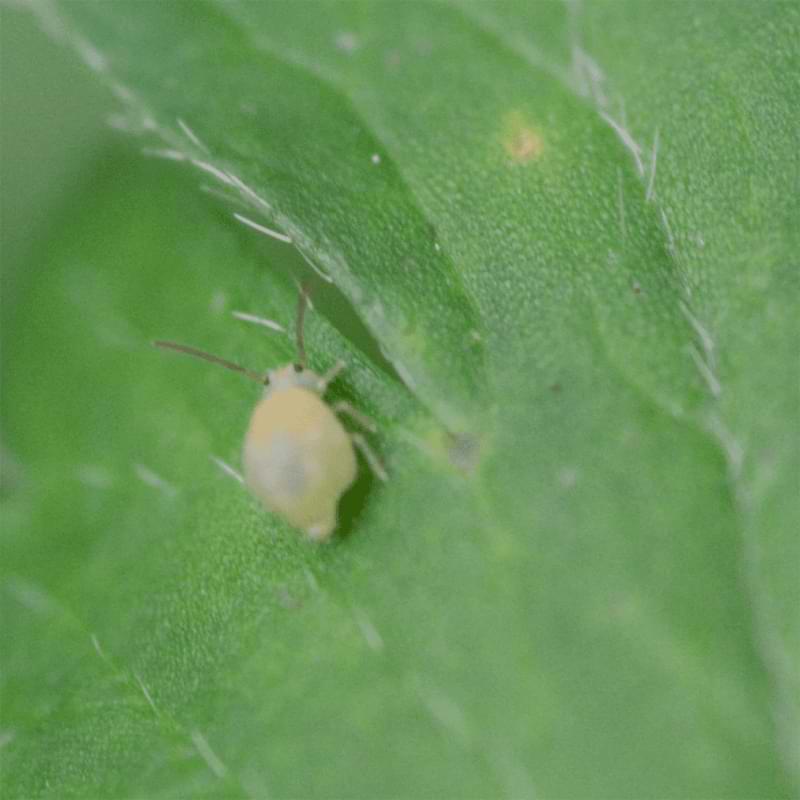The highly magnified image showcases a small bug perched on a green, pitted leaf, which might be part of a cacti or a shrub, although the extreme close-up makes it challenging to identify the plant precisely. The bug, possibly a stink bug or an aphid, is vividly green, with a prominent round abdomen. Its two dark antennae stretch out from its head, and it has six bent legs—three visible on the right side. Its black eyes are discernible despite the slightly fuzzy quality of the photograph due to the high magnification, which also reveals the leaf's intricate cell-like structure. The bug appears very tiny, emphasizing its minute size and delicate form.